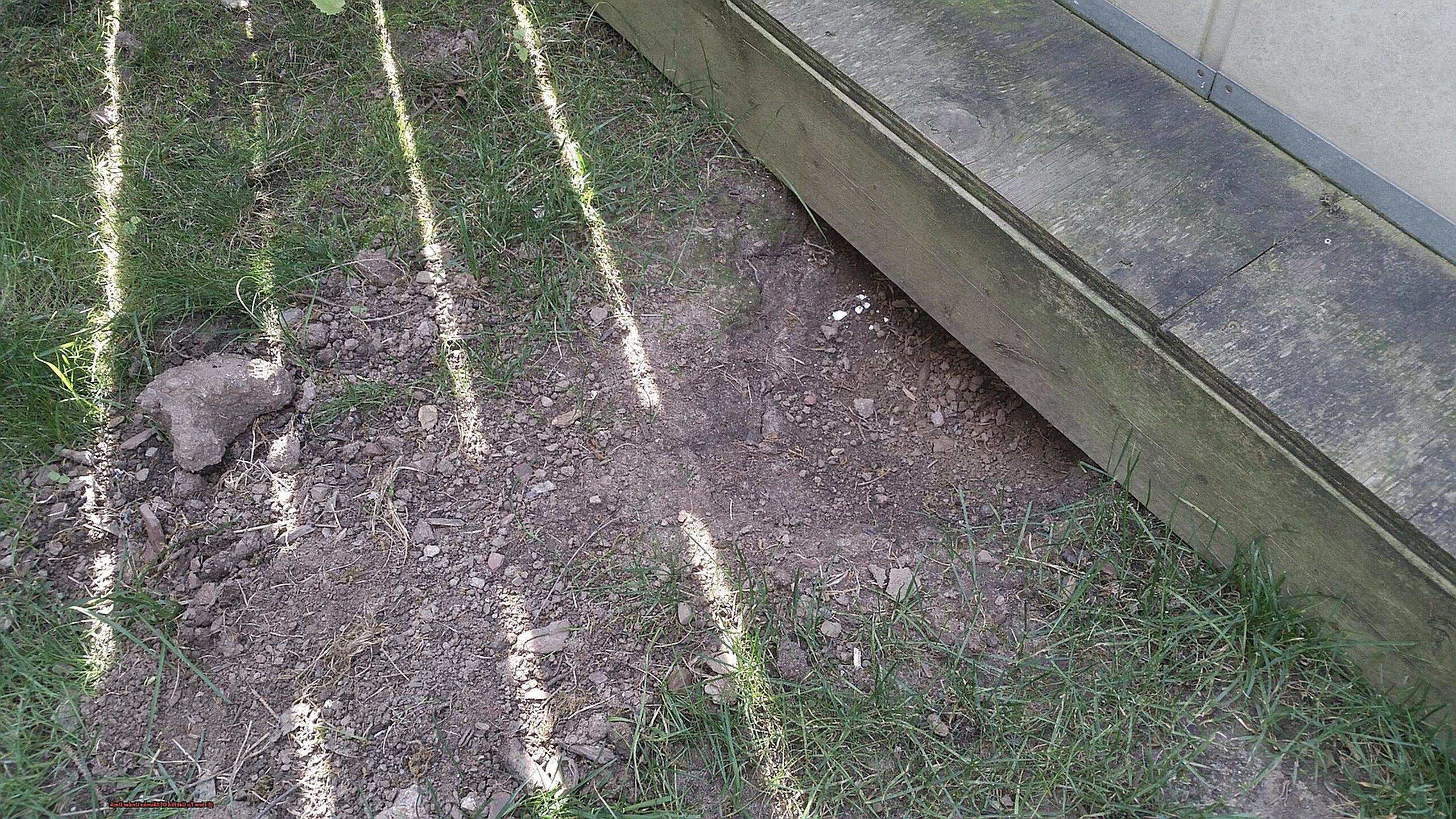The image depicts a weathered wooden frame lying on dry, dusty ground. This base frame appears to be part of a larger structure that is unseen but likely supported above it. Surrounding the frame is a fence, illuminated by sunlight that casts sharp shadows and reflections across the scene. At the corner of the wooden frame, a small hole has been dug, roughly resembling the shape of a wash pot, with scattered dirt suggesting animal activity. The frame shows signs of age and wear, with a green stain indicating past mowing and weeding, and the upper wooden structure exhibits blackened, aged timber. The overall ambiance is intriguing, especially considering the origin of the dug-out area and the interplay of sunlight and shadow through the fence slats.